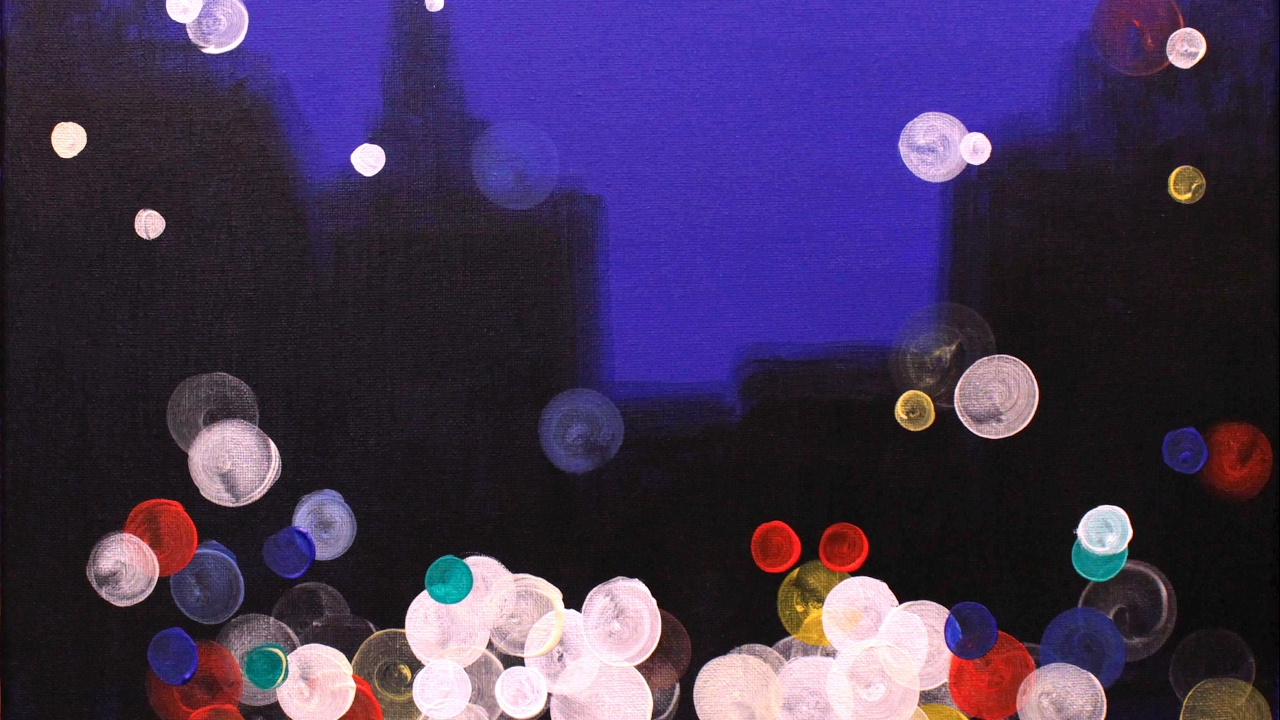This detailed abstract artwork showcases a horizontal rectangular composition set against a dark indigo or purple background. Dominating the foreground is a playful array of colorful circles or orbs, rendered in vibrant hues such as light pink, yellow, red, blue, teal, black, and even hints of beige and aqua. These orbs, which appear to have been painted with a finger or perhaps digitally created, lend a festive, almost sequin-like texture to the piece. Behind these orbs, a silhouette of buildings with taller towers and steeples emerges subtly in a dark, shadowy form. This silhouette is positioned towards the center-left, providing an intriguing contrast with the bright, scattered orbs that populate the lower portion of the image and sporadically float downward from the top. The absence of text keeps the focus squarely on the interplay of colors and shapes, contributing to the unique appeal of this visually striking and modern piece of art.